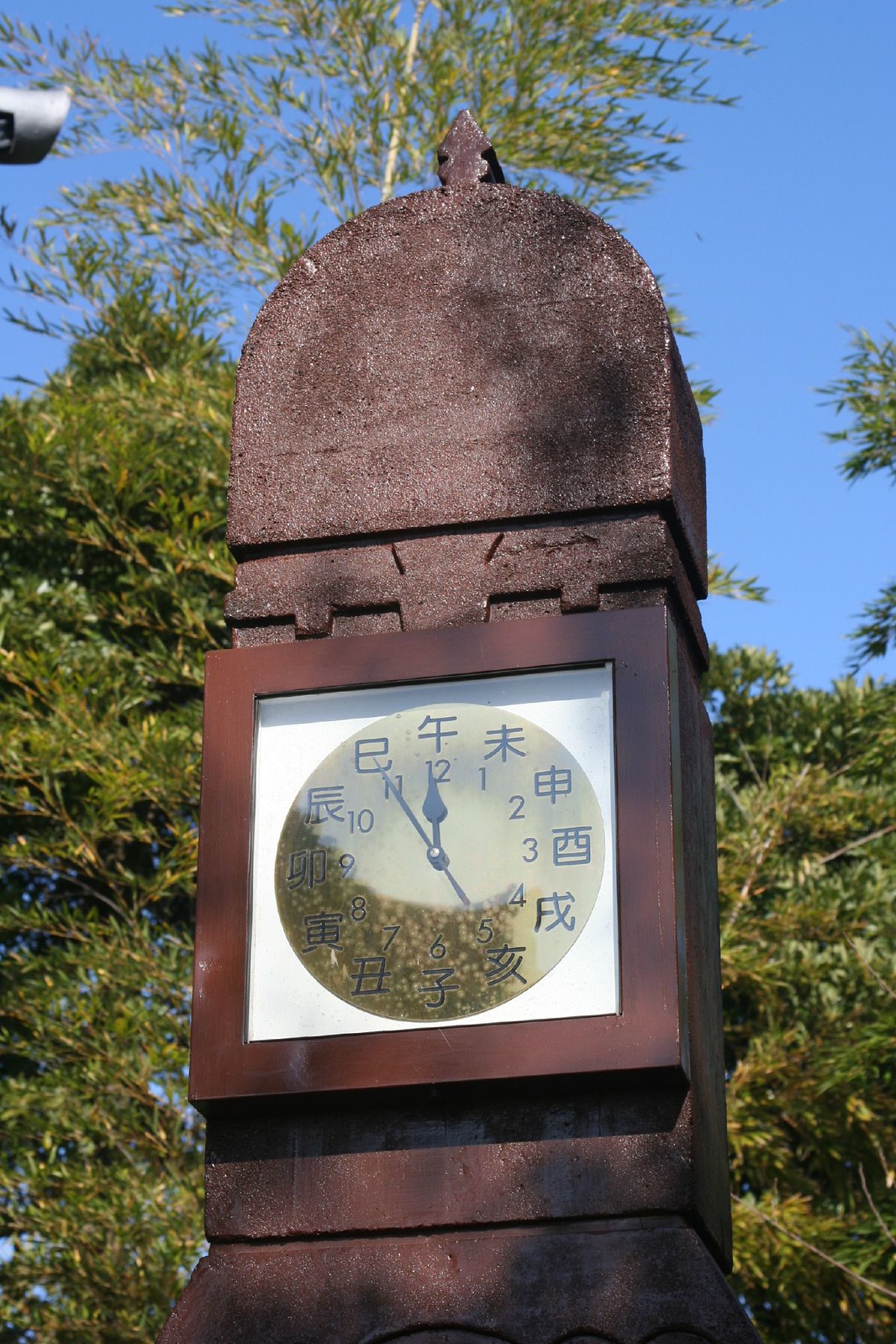This vibrant color photograph captures an unusual outdoor clock affixed to a refined stone monument amidst a clear blue sky and lush greenery. The monument, constructed from a brownish granite, features a smooth, curved top and stands as a dignified stone pillar. At the center of this pillar, a square wooden frame encloses a pristine white background, from which a classic round clock emerges. The clock face is adorned with traditional numerals from 1 to 12, encircled by intricate Chinese characters at the outer edge. Accentuated with elegant black hands, the clock displays the time as 11:55, while a slender, smaller hand points towards the number 5. The lower section of the clock's glass surface mirrors the surrounding trees, casting a gentle green reflection over the numerals and Chinese symbols, harmoniously blending the timepiece with its serene, natural environment.